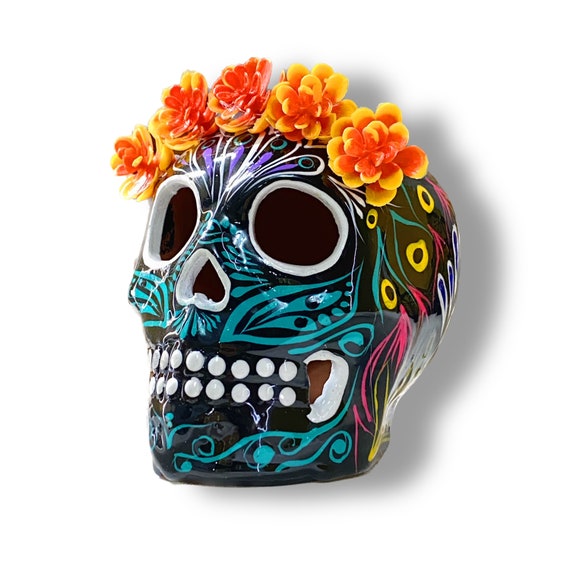The image depicts a Mexican Día de los Muertos (Day of the Dead) painted ceramic skull set against a white background with a digitally rendered shadow. The skull is oriented slightly to the left. It features a black base intricately decorated with various colors. The eye sockets, nose, and mouth are outlined in white, while white circles representing teeth line the mouth. A noticeable chip reveals the inner brown pottery on the right side of the mouth. The face is adorned with teal swirls near the nose and chin, along with yellow and pink accents on the sides, and purple patterns on the forehead. Crowning the top of the skull are five orange and yellow flowers, arranged in an arc, resembling succulents. The interior of the skull is a deep black, adding to its haunting yet festive appearance.